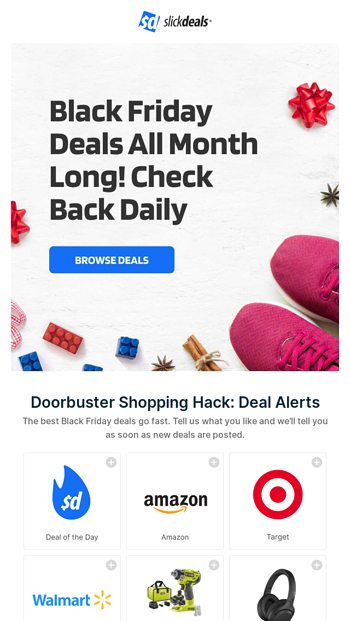The image is a screenshot from the Slick Deals app or the mobile browser version of the Slick Deals webpage, cropped to exclude the top navigation bar. The screenshot is a narrow vertical rectangle, indicative of a mobile device display. 

At the top, the Slick Deals logo is prominently centered on a white background. Below the logo, the background remains white, featuring a photo overlaid with text that reads, "Black Friday deals all month long, check back daily." Directly beneath this text is a blue button labeled "Browse Deals."

Following the promotional image, additional content on a white background provides further instructions: “Door buster shopping hack, deal alerts.” Subtext in smaller letters explains, “The best Black Friday deals go fast. Tell us what you like and we'll tell you as soon as new deals are posted.”

Below the text, there are six thumbnails arranged in a grid format. These thumbnails include icons representing various deal categories: Deal of the Day, Amazon, Target, Walmart, a set of tools, and a headset. Each thumbnail has a small gray X in the top right corner, presumably for dismissing the thumbnail.